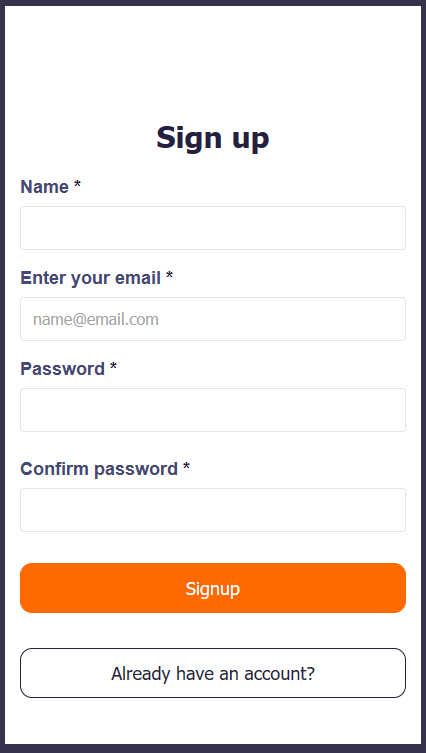The image captures a simple sign-up screen on a mobile device. The interface is designed with a clean, minimalist aesthetic, featuring a prominent, vertically aligned black rectangle outline against a white background, emphasizing the form. At the top of the screen, in bold black text, are the words "Sign Up."

Below the header, the form is organized into four required input fields, each marked with an asterisk. The first field is for the user's name, situated on the left-hand side of the screen. It features a very light gray text input box. Following this is a field for the user’s email, labeled "Enter your email." The text input box for the email has a faint gray border and displays the placeholder text "name@example.com" in light gray.

Continuing down the form, the third and fourth fields are for the password and the confirmation of the password, respectively. Both fields have light gray, empty text input boxes, indicating they are also mandatory.

At the bottom of the form, there is a bright orange rectangular button, stretching across most of the screen with rounded corners. The button stands out with the white text "Sign Up." 

Just beneath the sign-up button, there is a black outlined prompt with the text "Already have an account?" encouraging users who are already registered to take an alternate action. The overall design is straightforward, guiding the user through the necessary steps to create an account.